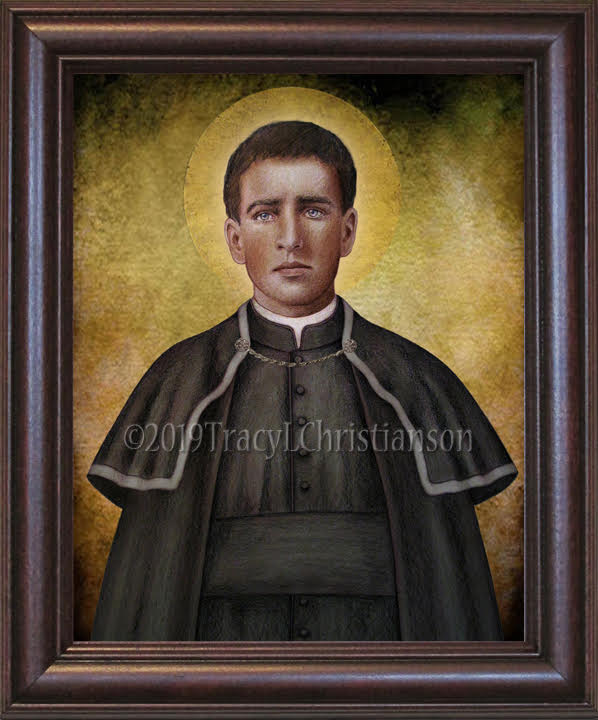The image is a detailed, drawn portrait of a young man dressed in attire reminiscent of a Catholic bishop or priest. He is depicted with a solemn gaze, looking into the distance, with striking blue eyes and short hair. The man is wearing traditional black religious clothes, including a priest's collar, a black shawl held by a chain and buttons, and a sash in the middle. Around his head, there is a golden halo, similar to those often seen in depictions of saints. The background of the portrait is predominantly gold, with some green and black patches adding depth. The portrait is enclosed in an intricate dark brown frame, featuring multiple layers with an outer, middle, and inner section. The artwork is copyrighted to 2019 by Trace L. Christensen, as indicated in the middle of the portrait.